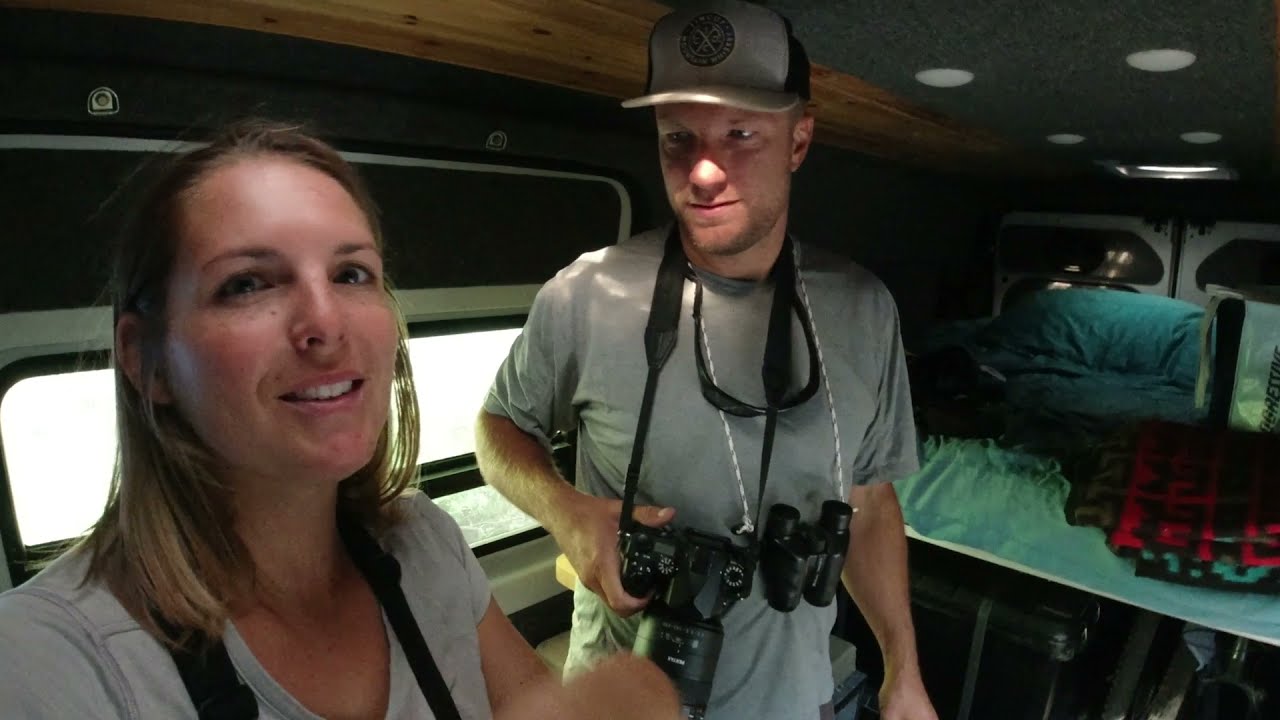In this detailed image, a man and a woman stand inside a vehicle that resembles a converted van or motorhome, set up as a living space. The man, positioned at the center, is wearing a gray t-shirt and a baseball cap with a white brim and logo, complemented by black sides. Around his neck, rests an impressive array of equipment: a sophisticated black DSLR camera with a strap, black binoculars hanging from a white and red rope-like strap, and sunglasses. The woman stands to his left, her shoulder-length blonde hair frames her smiling face, showcasing her visible teeth. She sports a white V-neck t-shirt and has a camera strap around her neck as well. 

Behind them, the interior includes darkened and small windows, a ceiling lined with gray fabric and inset lights, and wood paneling along the sides. The back of the vehicle features a makeshift bed, covered with blue sheets and pillowcases, and several colorful tied-up blankets. This bedding sits atop a storage area, with two white doors visible behind, likely part of the RV’s layout. Additional equipment and items, like a bag with black and white straps, are scattered around. The setting suggests they might use the vehicle for travel, photography, and outdoor activities such as bird watching.